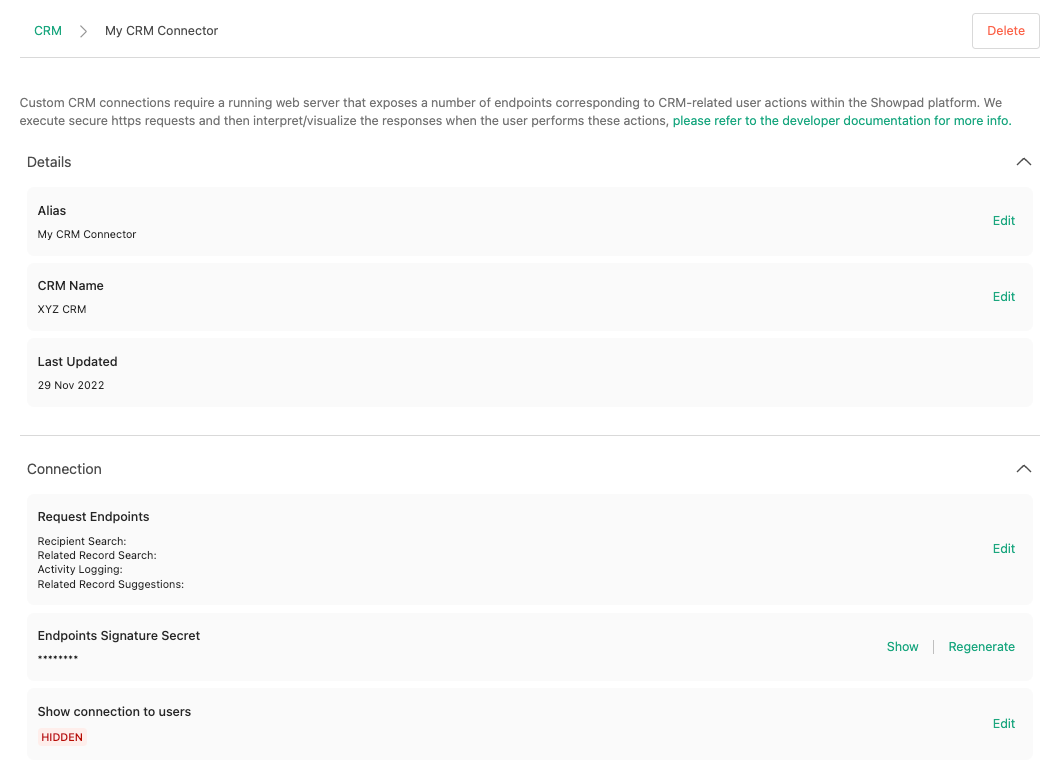The image depicts a dashboard interface for "My CRM Connector." 

At the top, the background is white, with the text "CRM" in green on the left side, styled to form the end of an arrow pointing right. The arrow transitions to gray, leading to the text "My CRM Connector" in black. 

Below, there is a gray rectangle with a red button labeled "Delete". A thin gray line traverses across the section. Following this, in gray text, it reads: "Custom CRM Connections require a running web server that exposes a number of endpoints corresponding to CRM-related user actions within a Showpad platform. We execute secure HTTPS requests and then interpret those visualized responses when the user performs these actions."

Further down, in green text, it instructs: "Please refer to the developer documentation for more info." Below this, in red text, the section is titled "Details", listing:
- Alias: My CRM Connector
- CRM Name: XYZ
- CRM RAS Updated: 2009
- OV: 2002

Another gray line separates the following section titled "Connection". This part details various endpoint requests:
- Request Endpoints
- Recipient Research
- Related Record Search
- Activity Login
- Related Record Suggestions
- Endpoint Signature Secret (with several asterisks below)

There is an option to "Show Connection to Users", marked by a light red rectangle and the word "Hidden" in red. 

Across from this, in green text, there are multiple "Edit" options listed, some accompanied by "Edit, Show" and "Regenerate" commands. The bottom of the image also features another "Edit" option in line with the others.